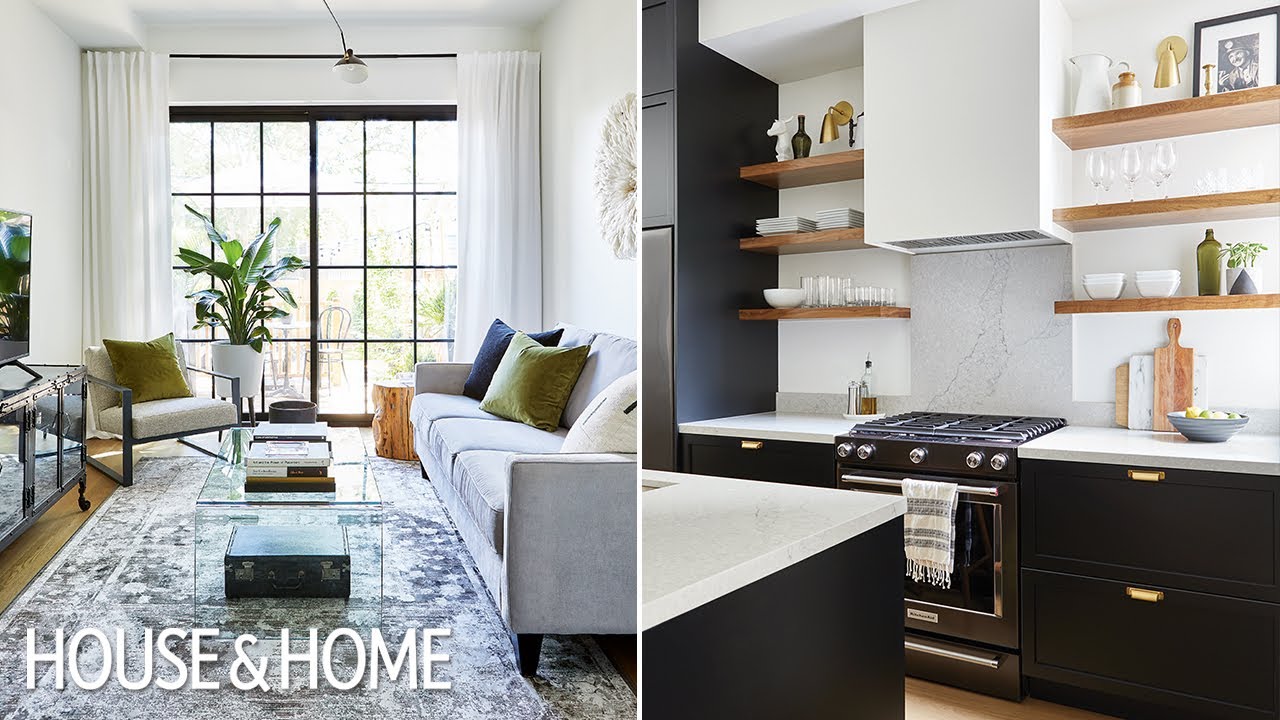This image from House and Home magazine features a detailed view of two rooms in a home, shown in a landscape orientation. On the left side, there is a living room characterized by a large, blue and white rug on a hardwood floor. The centerpiece is a blue couch adorned with blue, green, and white pillows, positioned along the right-hand side of the room. A clear glass coffee table with books on it sits in front of the couch, and underneath it, there is a suitcase. Adjacent to this, a unique tree trunk side table adds a rustic touch. The backdrop of the living room is dominated by a large, black-framed sliding patio door adorned with white curtains, opening to a view outside where a chair can be seen. In the left corner, there is a small upholstered chair with wrought iron armrests, white fabric, and a green pillow, complemented by a green potted plant in a white vase. Additionally, a glass console table holding a television is positioned against the left-hand wall. 

On the right side, the image showcases a modernized kitchen with a blend of contemporary and functional design elements. The kitchen features white countertops, a marble backsplash, and black cupboards. Above, open wood shelving displays an assortment of bowls, glasses, and pictures. A standout appliance in the kitchen is a gas stove, set amidst wooden and marble cutting boards that rest on the countertops. The space also includes a bowl of fruit, contributing to a vibrant and homely atmosphere. The bottom of the image is captioned with the text "House and Home" in white.